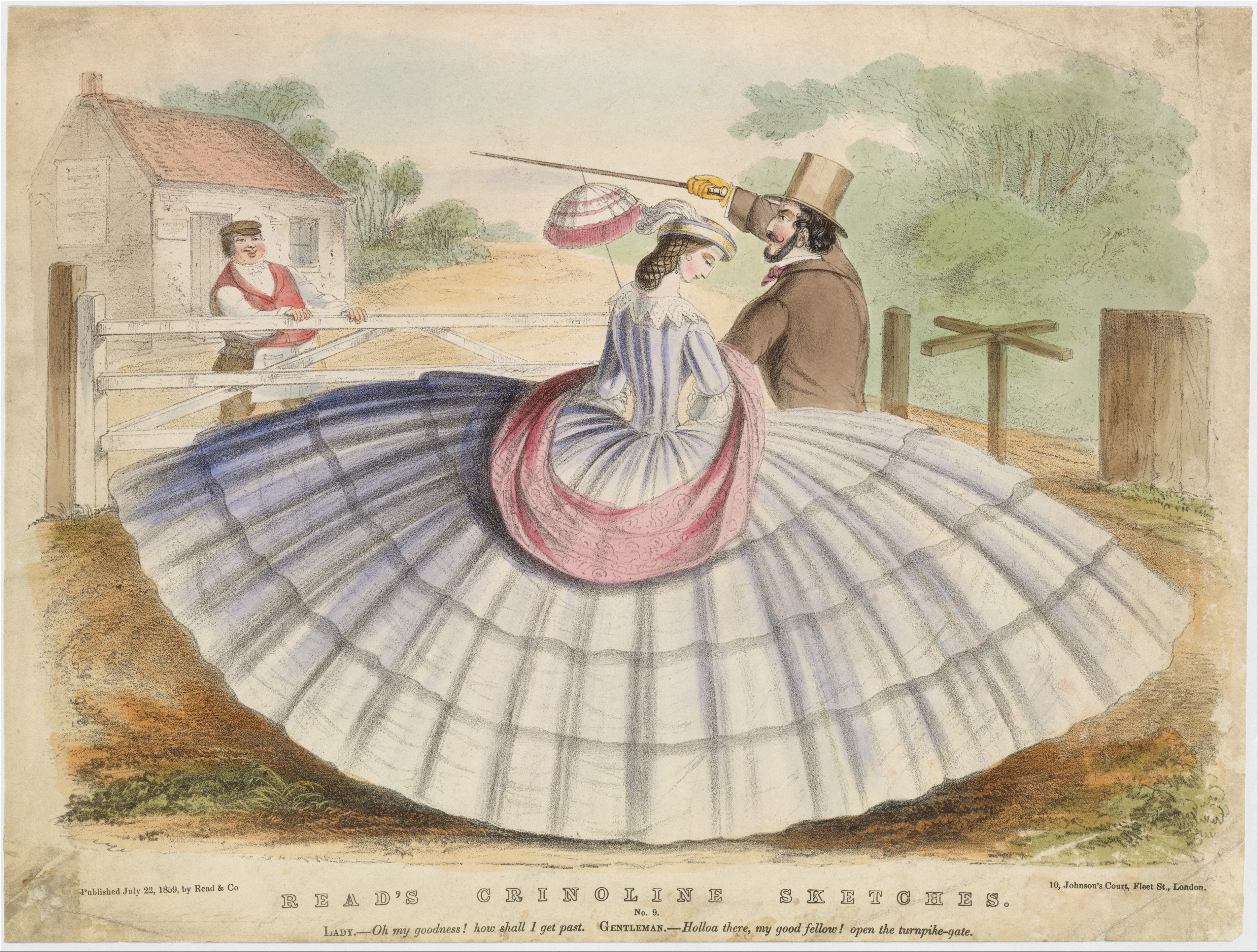The illustration or painting captures a rural countryside scene with a central focus on a woman dressed in an ornate, hoop-skirt gown that frills out dramatically, creating an exaggerated, umbrella-shaped silhouette. Her gown, in shades of grayish-white with a checkered pattern, features a pink sash at the waist. The woman is turned away from the viewer, gazing downwards to the right side of the image. She carries a parcel that matches her outfit, adorned in white, gray, and pink.

Standing to her left is a man in a brown suit and hat, holding a stick that extends to a small parasol at the end, humorously attempting to shade the woman despite the distance created by her grandiose skirt. The man, sporting a beard and mustache, points towards the left side of the image.

In the backdrop, separated by a white wooden fence, is another woman dressed in red and white, smiling and engaged in conversation with the couple. She stands in front of a white house with a sloped red roof. The scene is set along a long path flanked by trees, emphasizing the tranquility of the countryside. Text at the bottom of the image reads "Brad's crinoline sketches," suggesting the theme revolves around the extravagant fashions of a bygone era.